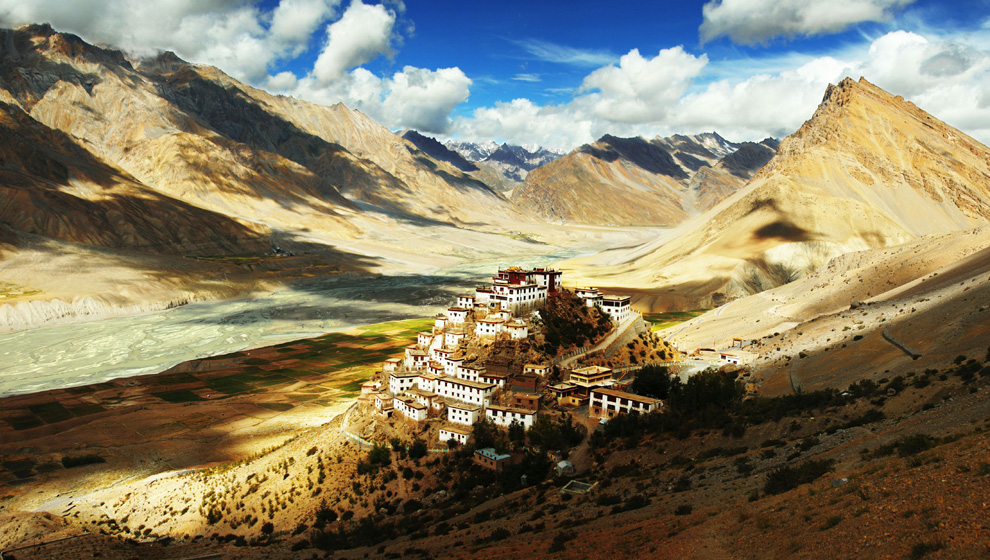The image showcases a large, white complex of buildings situated at the heart of an arid landscape. These structures are intricately connected, forming a small town with numerous windows. Atop the complex, a small, dark brown building stands out dramatically against the lighter hues. Surrounding this urban cluster, the desert terrain presents itself with light brown, sandy mountains extending to the left, right, and far into the distance. The barren land below contrasts sharply with the pockets of vibrant, green trees, lush with foliage. The sky above is a clear, vivid blue, dotted with fluffy, white clouds that float serenely, adding a dynamic elegance to the scene. Sunlight bathes the upper half of the image, casting a warm glow, while the lower right corner remains cloaked in a large patch of shade, creating a stark play of light and darkness in the composition.